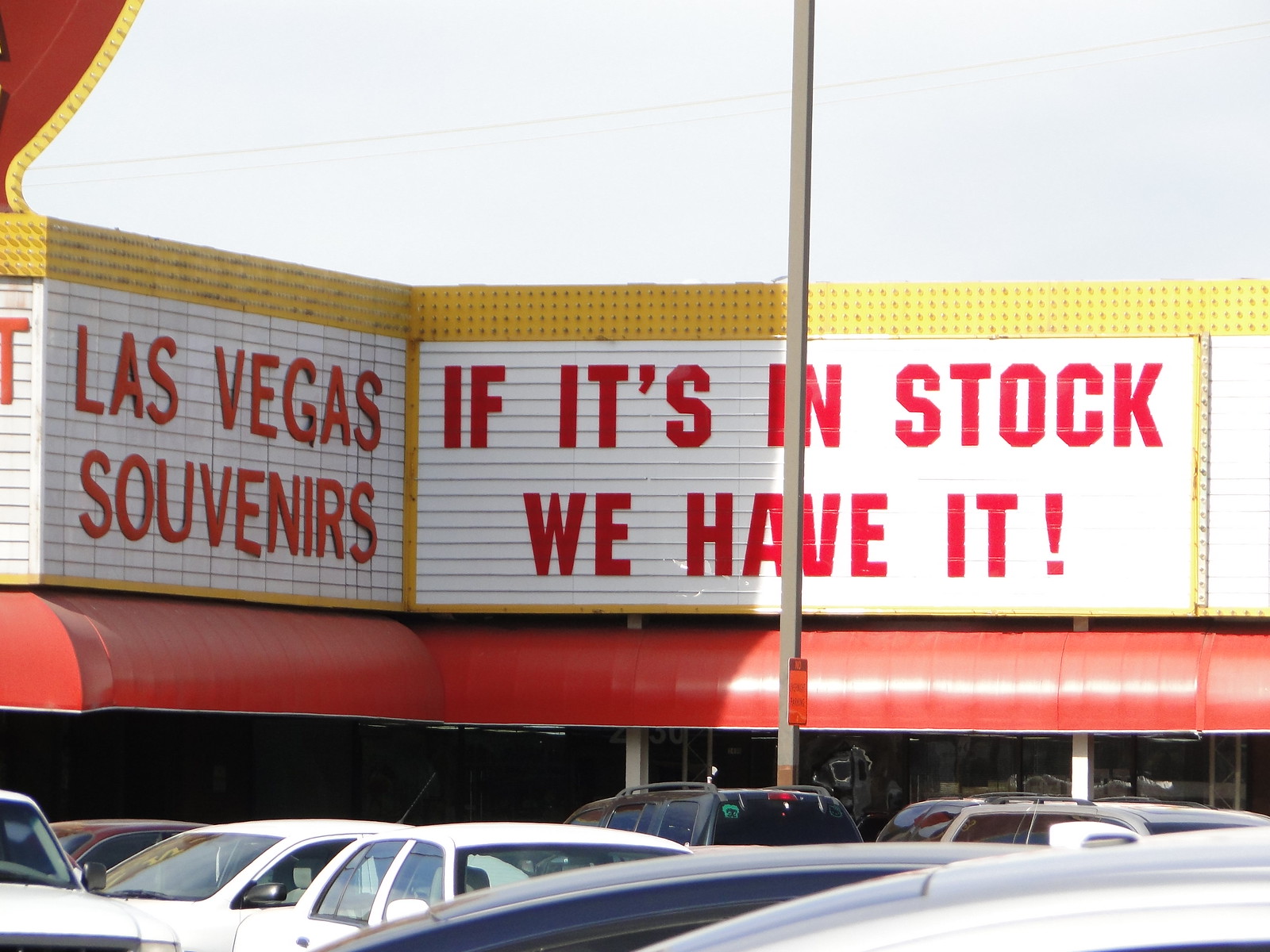This is an outdoor photo of a sign attached to a business, taken from a parking lot looking toward what appears to be a shopping center in Las Vegas. The prominently displayed white marquee sign features large, capitalized red letters in a sans-serif font that read "Las Vegas Souvenirs. If it's in stock, we have it!" The sign is mounted above a red awning which stretches across the building facade, beneath which there is a bank of windows that appear shadowy and obscure. In the foreground, numerous cars are parked in the business's lot, with only the tops and hoods visible. The scene also includes a gray metal lamppost that partially obstructs the view of the sign. The sky has a stark, almost white appearance, likely due to increased contrast, although the weather suggests a typical warm and sunny day in Las Vegas. The building itself is older in style, reminiscent of a traditional strip mall.